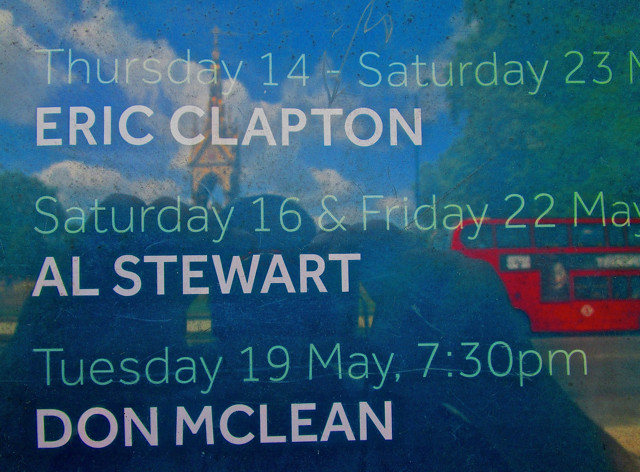This image features a shiny, slightly dirty sign displayed on a window, reflecting a sunny day with white clouds, trees, a church steeple, and a red double-decker London-style bus. The reflection also shows a person with a camera held to their face, obscuring their identity. The sign lists several events: "Thursday 14 through Saturday 23 Eric Clapton," "Saturday 16 and Friday May 22nd Al Stewart," and "Tuesday 19 May 7:30 p.m. Don McLean." The surface of the sign shows noticeable splotches and scratches, adding to the scene's lived-in feel.